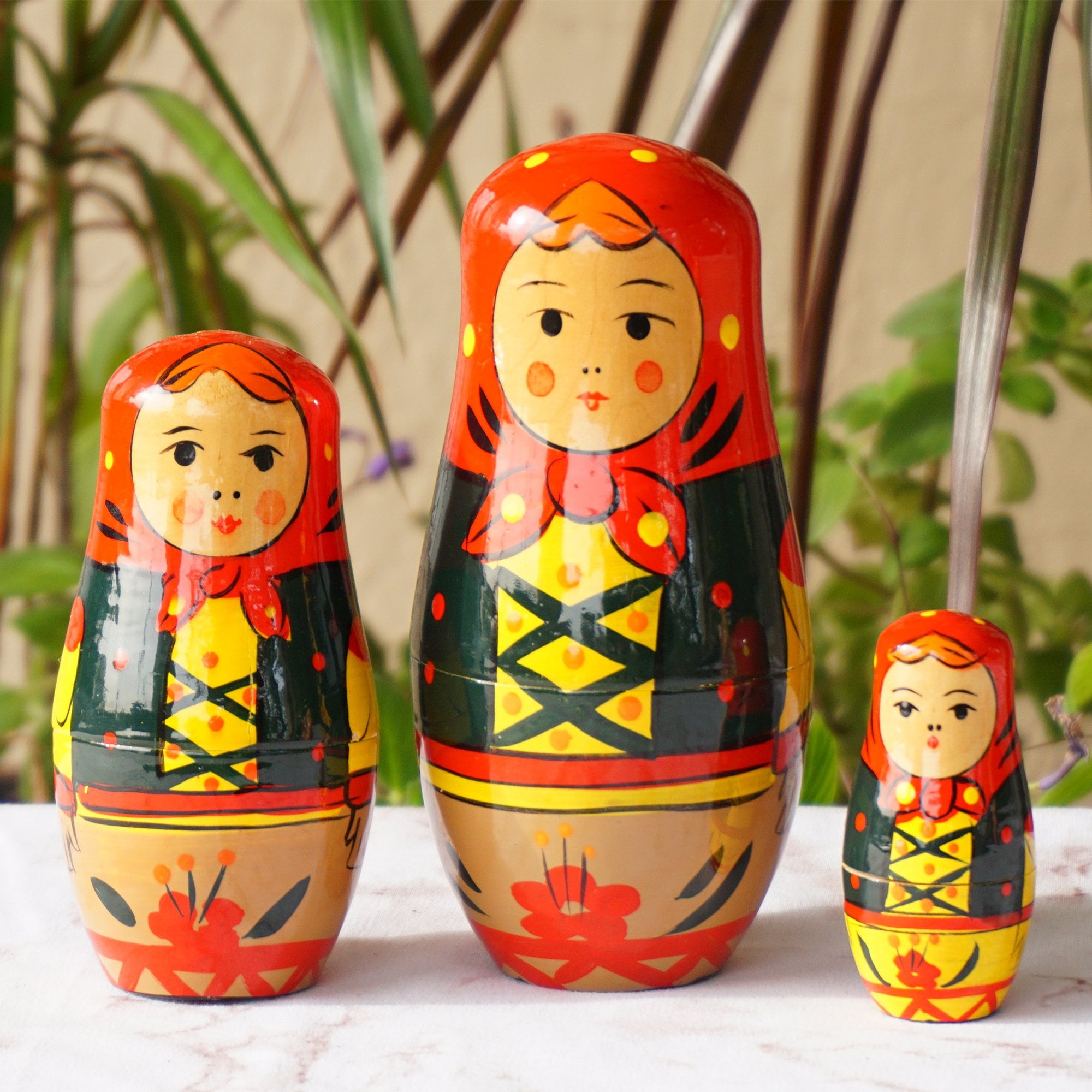The photograph features a set of three traditional Russian nesting dolls, or Matryoshka dolls, arranged on a windowsill adorned with palm leaves in the background. Each doll, fashioned out of wood and meticulously hand-painted, fits inside the next larger doll, creating a fascinating nested design. They all feature identical, simple yet charming faces reminiscent of a Kewpie doll, complete with one rosy red cheek and another tan cheek. The dolls are topped with bright red babushkas detailed with green ornamentation and showcase orange hair peeking through. They wear dark green vests laced at the front, over yellow tops, and are adorned with floral and dotted patterns. The largest doll is centrally placed with the medium-sized doll on the left and the smallest on the right, all standing upright on a piece of granite, emphasizing their intricate traditional artistry.